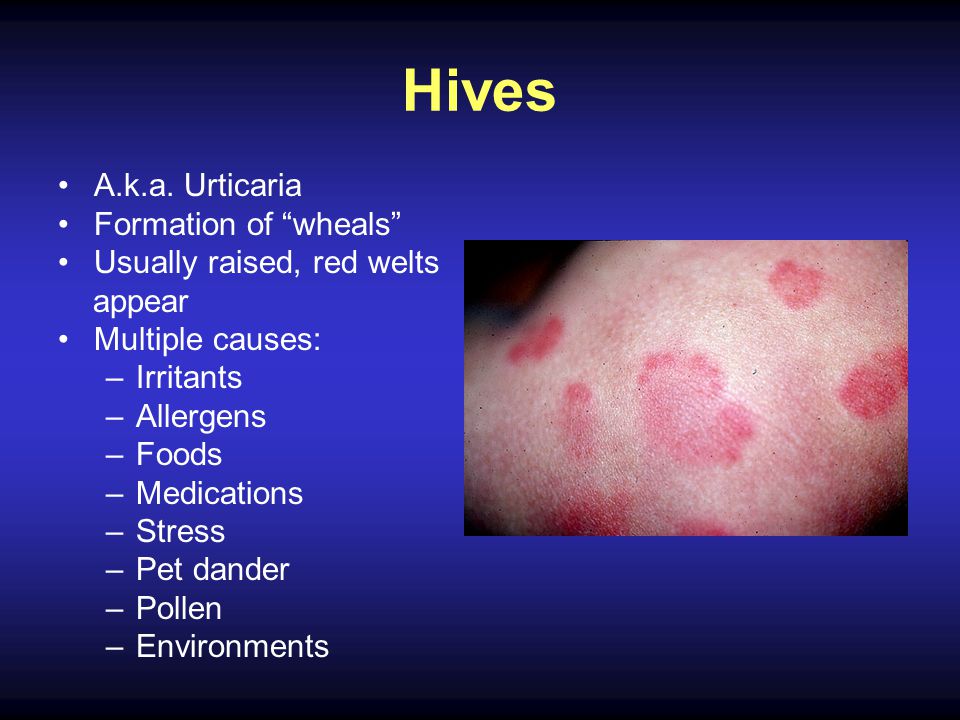This is a detailed PowerPoint slide used for a medical presentation. The slide features a background with a blue to black gradient. At the top, the title "Hives" is prominently displayed in yellow text. On the right side of the slide, there is a close-up photograph depicting red patches of hives on someone's skin, which appears to be a hand. On the left side, there are informative bullet points written in white text that explain the condition: 

- a.k.a. urticaria, spelled U-R-T-I-C-A-R-I-A
- Formation of wheals (spelled W-H-E-A-L-S)
- Usually raised, red welts appear
- Multiple causes or irritants:
  - Allergens
  - Foods
  - Medications
  - Stress
  - Pet dander
  - Pollen
  - Environmental factors

The slide comprehensively outlines the symptoms and potential triggers of hives, making it a useful educational tool.